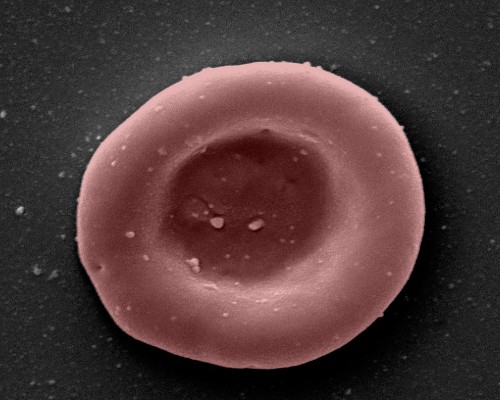The image depicts a circular, donut-shaped object with a concave center, prominently situated against a textured black background. The background varies from lighter to darker shades of black and features tiny white specks and grain-like elements scattered throughout. The central object, resembling a blood platelet or a red blood cell, exhibits a gradient coloration; its outer edges are a light maroon or muted red, transitioning to a much darker brownish-red in the center. This microscopic image, viewed from above, captures the fine details and textures of the object and the surrounding speckled background, creating a stark contrast that highlights the central feature.